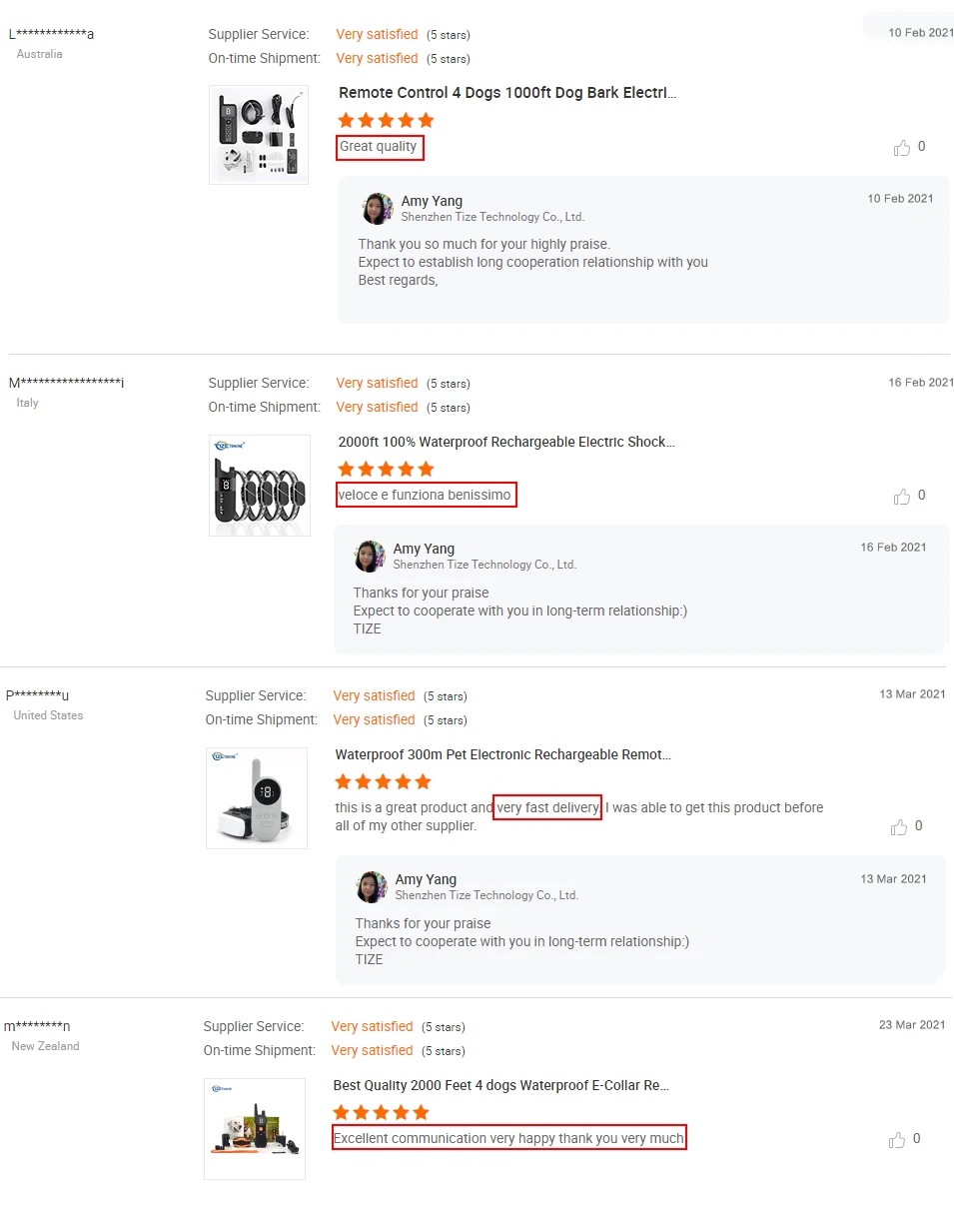**Product Reviews Page Description**

The image features a webpage displaying multiple product reviews. Each reviewer’s identity is partially masked, showing the initial and final letters of their username, with asterisks in between, along with their country of origin.

1. **Reviewer from Australia:**
   - **Ratings:**
     - Supplier Service: Very Satisfied (5 stars)
     - On-time Shipment: Very Satisfied (5 stars)
   - **Product:** Remote Control for Dogs, 1,000-foot Range, Anti-Bark.
   - **Review:** 5 stars, "Great Quality."
   - **Reply from Amy Yang:** "Thank you so much for your high praise. We look forward to establishing a long-term cooperation relationship with you. Best regards."

2. **Reviewer from Italy:**
   - **Product:** 2,100% Waterproof Rechargeable Electric Shock Collar.
   - **Review:** 5 stars, written in Italian.
   - **Reply from Amy Yang:** "Thanks for your praise. We expect to cooperate with you in a long-term relationship."

3. **Reviewer:**
   - **Product:** Waterproof 300-meter PET Rechargeable Remote Dog Training Collar.
   - **Review:** "This is a great product and very fast delivery. I was able to get this product before all of my other suppliers."
   - **Reply from Amy Yang:** "Thanks for your praise. Expect to cooperate with you in a long-term relationship."

4. **Reviewer:**
   - **Product:** Best Quality, 2,000-foot Range, Four-Dog Waterproof E-Collar.
   - **Review:** 5 stars.

Each product showcased in the reviews is accompanied by a photograph, enhancing the visual representation of the items being discussed. The replies from Amy Yang maintain a consistent tone, thanking the reviewers and expressing a desire for continued business collaboration.